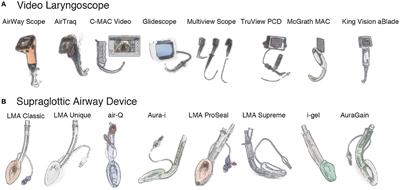The image is a detailed color illustration infographic in landscape orientation, depicting various types of medical devices used for airway management. It features two rows of color illustrations against a white background, each labeled with black text headings. The top row (labeled A, "Video Laryngoscope") includes eight closely-aligned illustrations: Airway Scope, Airtraq, C-MAC Video, Glidescope, Multiview Scope, TrueView PCD, McGrath MAC, and King Vision aBlade. The bottom row (labeled B, "Supraglottic Airway Device") captures another eight devices with larger text headings: LMA Classic, LMA Unique, AirQ, RRI, LMA ProSeal, LMA Supreme, iGel, and AuraGain. The illustrations, done in pastel colors and somewhat crude in detail, collectively emphasize the diverse range of these critical medical tools.